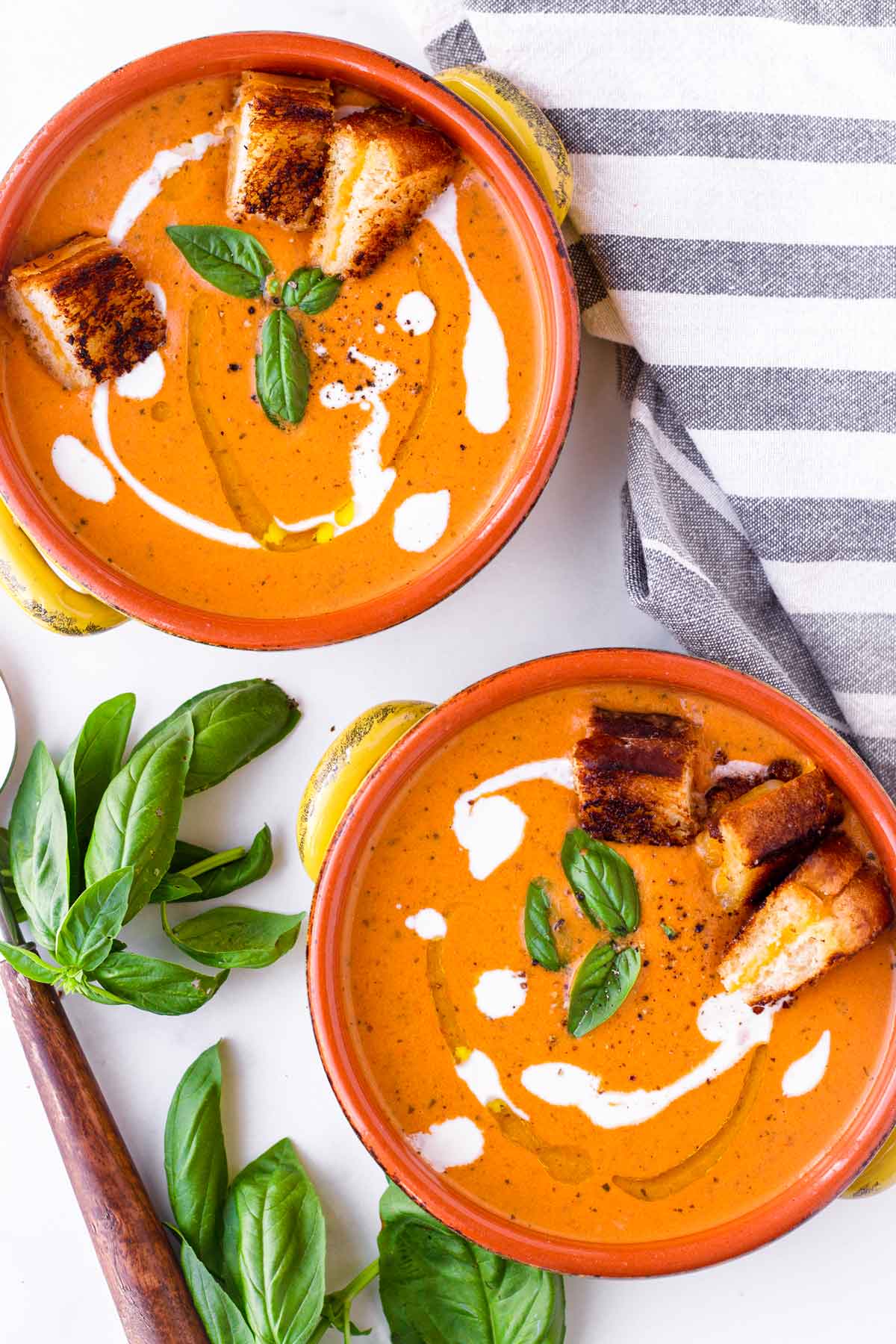This professional food photography showcases two orange bowls of a tomato-based soup, each artfully garnished with basil leaves, a drizzle of cream, and pieces of toasted bread. The composition is set against a pristine white background, with a rustic wooden-handled spoon positioned on the bottom left and a piece of napkin fabric in the top right corner. The bowls are thoughtfully staged, one in the bottom right and the other slightly overlapping it towards the top. The photograph, taken from a top-down perspective, features vibrant hues of orangish-tomato, greens, creamy whites, cheesy yellows, grays, blacks, and browns, all enhanced by professional lighting that suggests a studio setting. The soup is also seasoned with pepper and a hint of olive oil, highlighting the meticulous attention to detail in this culinary presentation.